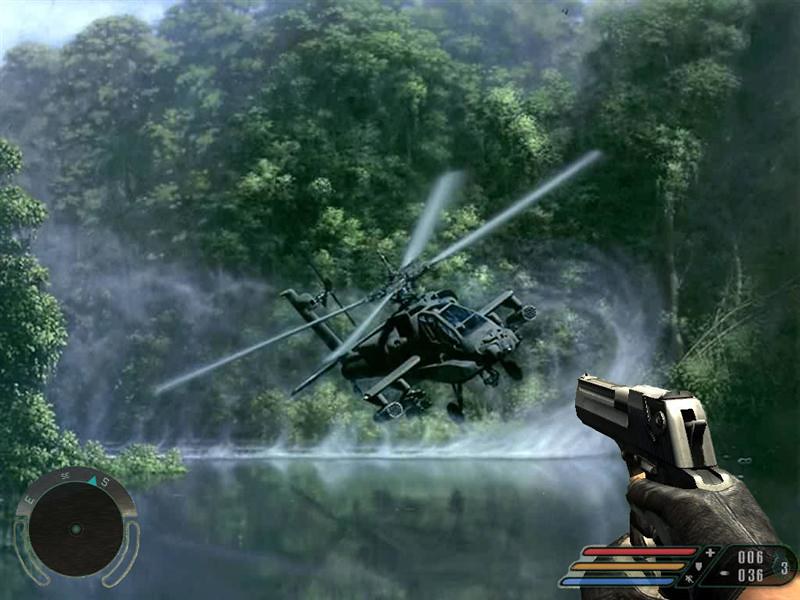This screenshot from a video game captures an intense moment where a player, represented by a black-gloved hand holding a silver pistol, aims at a military-style helicopter flying low over a lake. The helicopter, equipped with guns under each wing, stirs up water vapors as its blades appear stationary in the still image. Surrounding the lake is a lush, green forest that resembles a rainforest, with the trees reflecting vividly in the water below. On the gaming HUD, located at the bottom right corner of the screen, there are three colored bars: a red health bar, a yellow defense bar, and a blue skill or mana bar. Accompanied by white text, the display indicates there are 6 bullets in the magazine and 36 in the inventory, with an additional white number 3 to the right of these bars. Additionally, the bottom left corner of the screen features a black and gray compass, showing the player’s orientation.